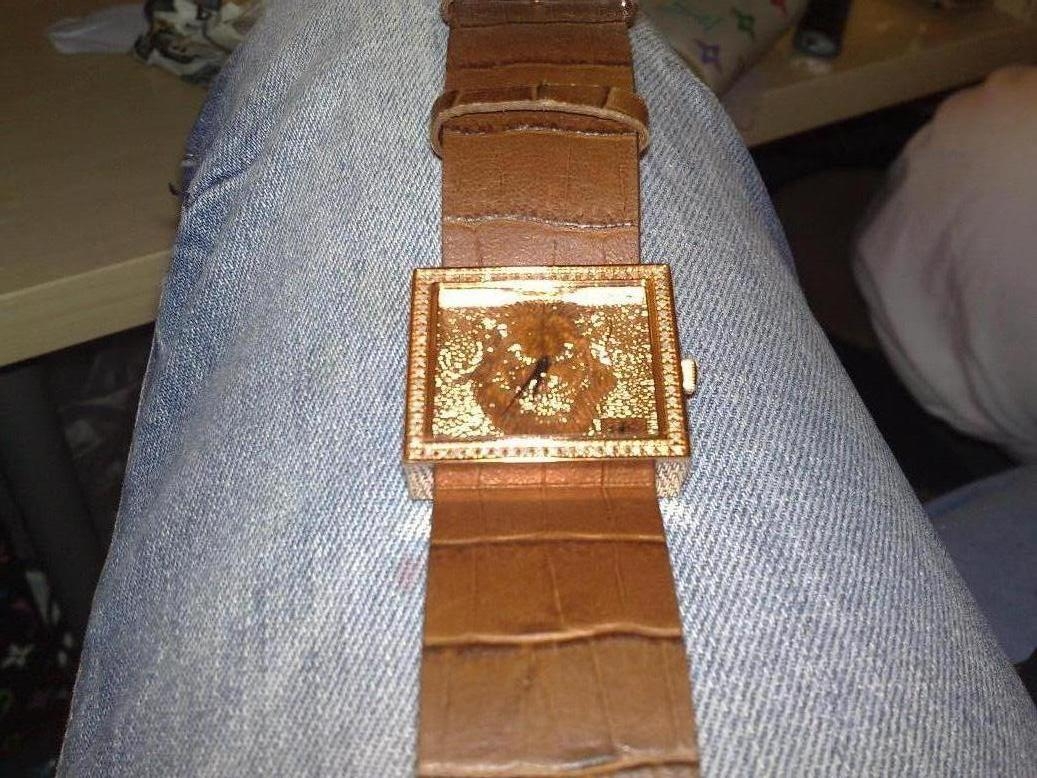This real-life photo features a detailed scene centered around a prominently displayed wristwatch. The watch is laid across the thigh of a person who is wearing a pair of faded, light blue denim jeans. Occupying about 60 to 70% of the frame, the person's denim-clad leg dominates the image, with the wristwatch meticulously positioned on top. The watch itself boasts a light brown leather strap that extends from the top to the bottom of the image, wrapping around a square, gold-plated case. 

The square face of the watch is particularly striking, adorned with intricate gold leaf embellishments that form the image of a lion's face and mane. The dark brown center of the watch face lacks numerical markers, featuring black hands instead. A small turn knob is visible on the right side of the case, hinting at its functional design.

In the background, a light brown wooden table is partially visible. On this table are a Louis Vuitton wallet and a Bic lighter, both positioned at the edge of the frame. Additionally, part of a white cloth or bag is discernible on the right side of the photo, adding another layer of depth to the scene. The detailed imagery and composition highlight the watch's ornate design against the casual backdrop of denim and everyday objects, creating an intriguing juxtaposition.